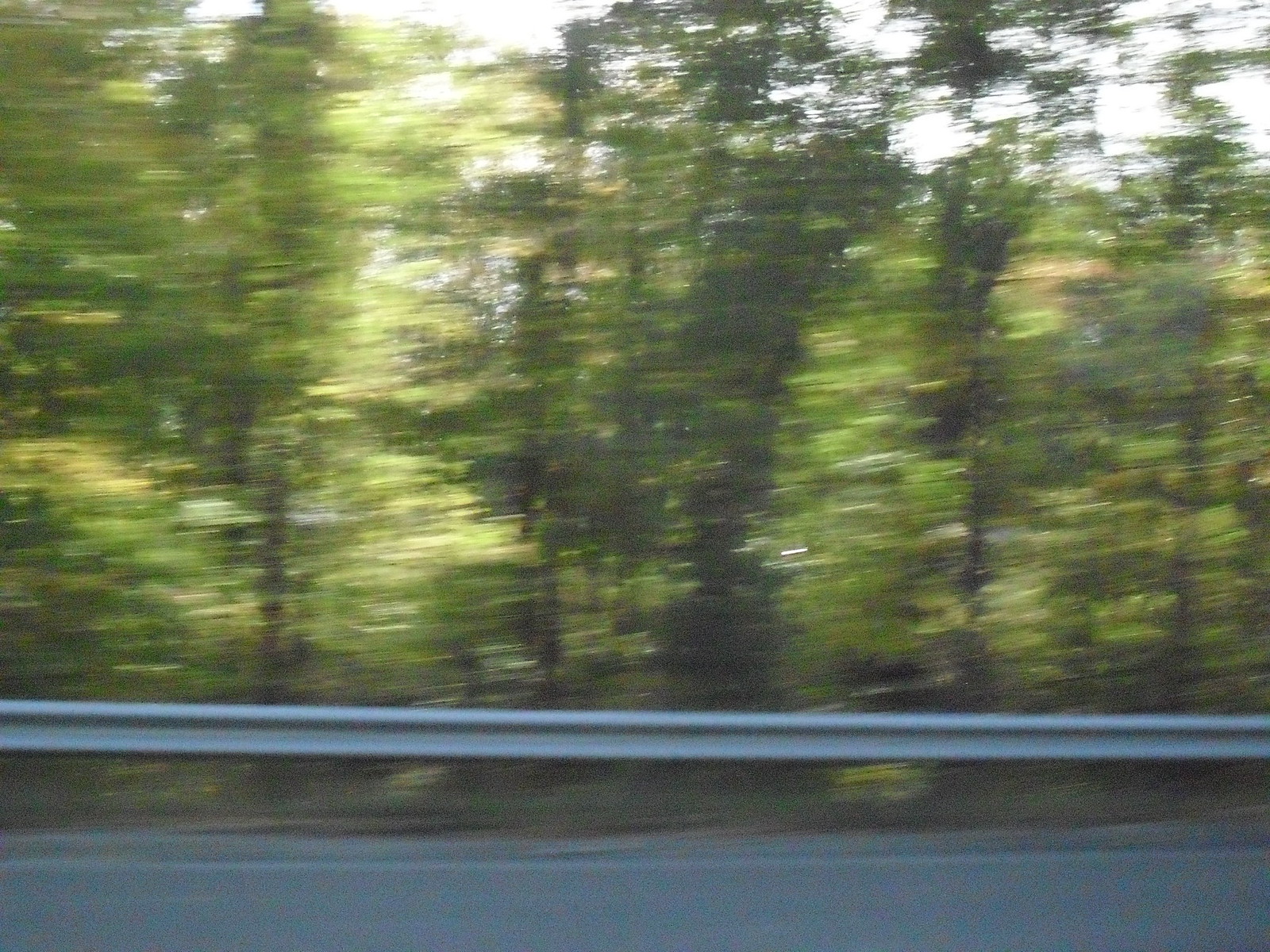The photograph depicts a scene from a moving vehicle, characterized by its motion blur. In the foreground, a gray road runs horizontally, bordered by a metal guard rail. Behind the guard rail, a dense, forested area with numerous tall, thin trees stretches out, thick with green leaves. The daylight scene has an overexposed sky, with sunlight filtering through the trees, casting reflections down to the ground. The image captures the essence of motion and the serenity of a wooded landscape.